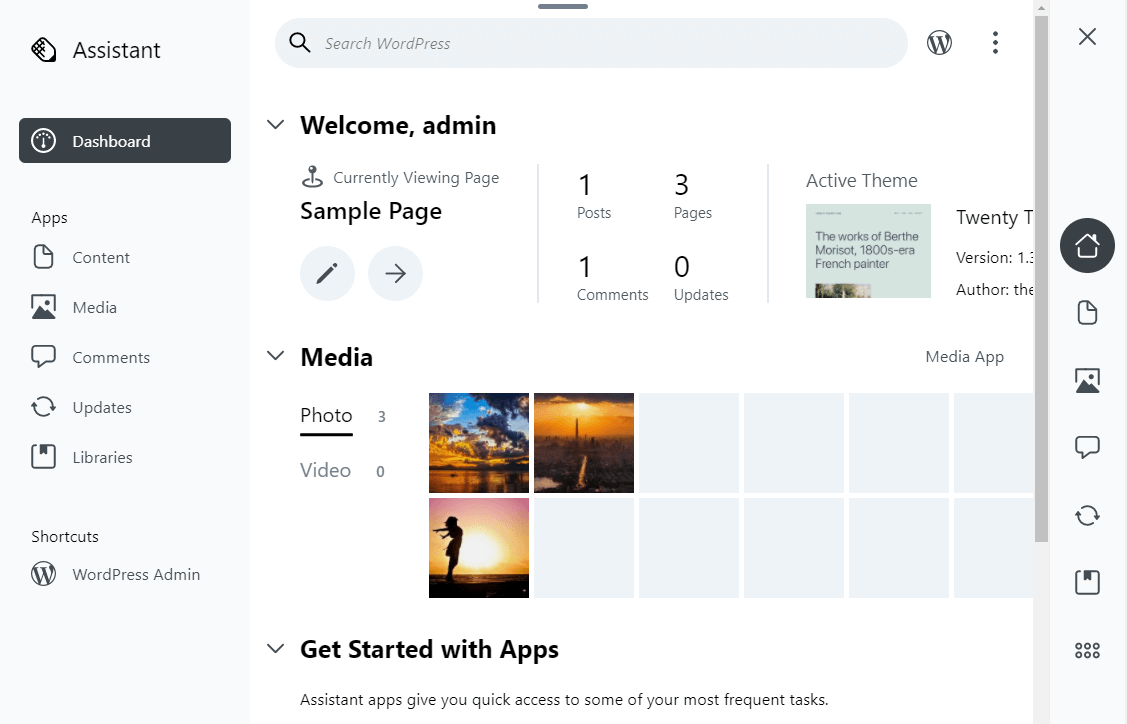On this page, we are viewing a post on a WordPress site. There is a prominent search bar, labeled "Search WordPress." This indicates that the platform being used is indeed WordPress, a widely known website development service that allows users to create and manage their own websites for a fee. 

The main section of the screen welcomes the admin with the message "Welcome Admin." It also provides access to the homepage and media library, which currently contains only three photos since the site is still in its early stages. On the left, a sidebar assistant displays various options available to the user, starting with the dashboard, which is highlighted in a dark blue/grey color, indicating it's the current selection.

Other available options in the sidebar include content, media, comments, updates, and libraries. Additionally, there are shortcuts to WordPress admin support for troubleshooting any technical issues that may arise while using the platform. This detailed and customizable interface is geared towards providing site administrators with a robust suite of tools for managing their WordPress site.